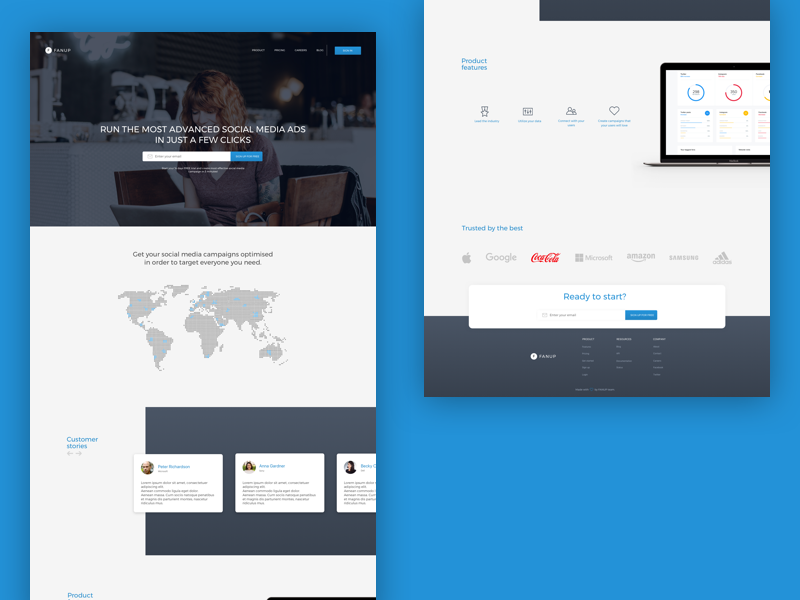A promotional graphic set against a blue background features a woman using a laptop. The laptop's screen displays an advanced social media advertising platform with a user-friendly interface that enables campaigns to be crafted and optimized with ease. A map overlay indicates targeted reach capabilities. 

Three white rectangles on a black background showcase customer testimonials complete with profile pictures, names, and brief information snippets. These rectangles feature images of a man and two women. 

Adjacent to these testimonials, product features are highlighted with four corresponding icons, detailing the key functionalities of the platform. 

The graphic further emphasizes the platform's credibility by showcasing logos of esteemed companies, such as Google, Coca-Cola (in red), Microsoft, Amazon, Samsung, and Adidas. 

At the bottom, a black section lists additional details in white text, with a call-to-action message "Ready to start?" prominently displayed in blue.